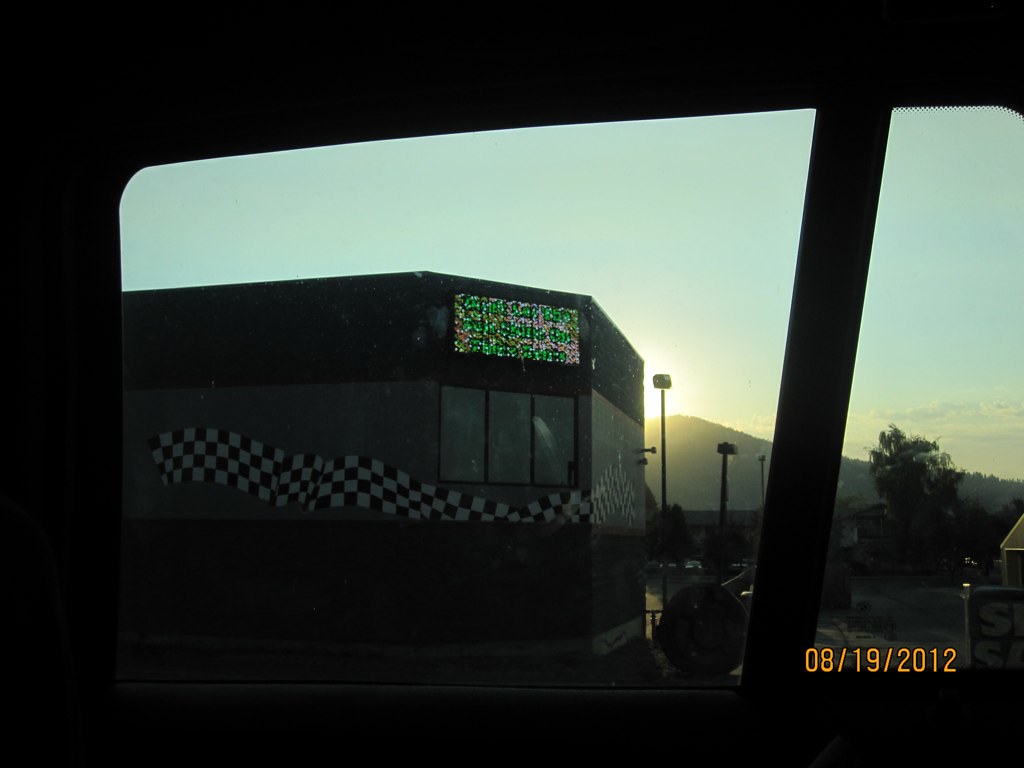In this dimly lit photograph, taken from the window of a vehicle, we observe the front facade of an oblong-shaped building adorned with a black and white racing stripe banner along its side. Above the windows, a sign illuminated with green and white lights stands out against the building's exterior. In the far distance, the sun hovers just above a hill, its light barely piercing through the horizon, suggesting either dawn or dusk. The sky features a diffuse grayish-blue hue, punctuated by a few scattered clouds. The timestamp, displayed prominently in orange at the lower right corner, marks the date as 08-19-2012.